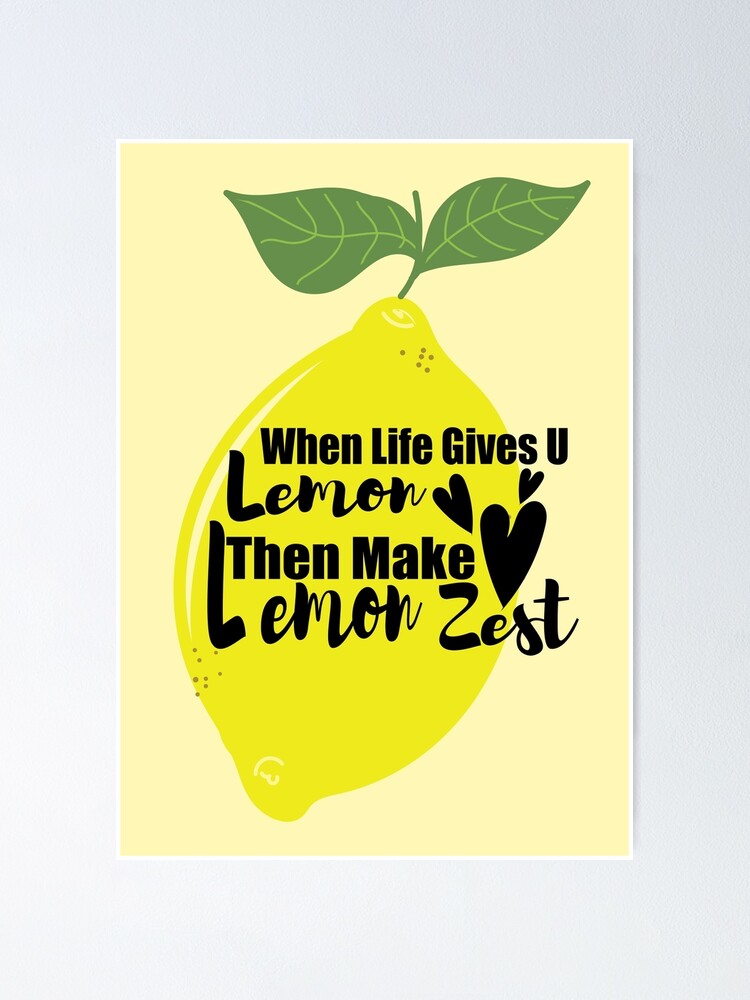This is a piece of homey artwork reminiscent of what might be found at a dollar store. The vertically oriented image showcases a stylized lemon with two green leaves at the top, drawn on a light yellow background, possibly a thin canvas or paper print, set against a creamy white matte mount. The cartoonish yellow lemon features a shine mark on its left edge, suggesting luster and freshness. Written across the lemon in quirky, shifting black fonts is the phrase: "When life gives you lemons, then make lemon zest." The words "When life gives you" are in a thick, blocky font, while "lemons" and "lemon zest" are rendered in a careless, cursive script. Scattered around the text are several narrow black hearts, adding a whimsical touch to the design. The entire artwork comes across as a simple, cheerful piece with no additional text or signature, highlighting its lighthearted and motivational message.